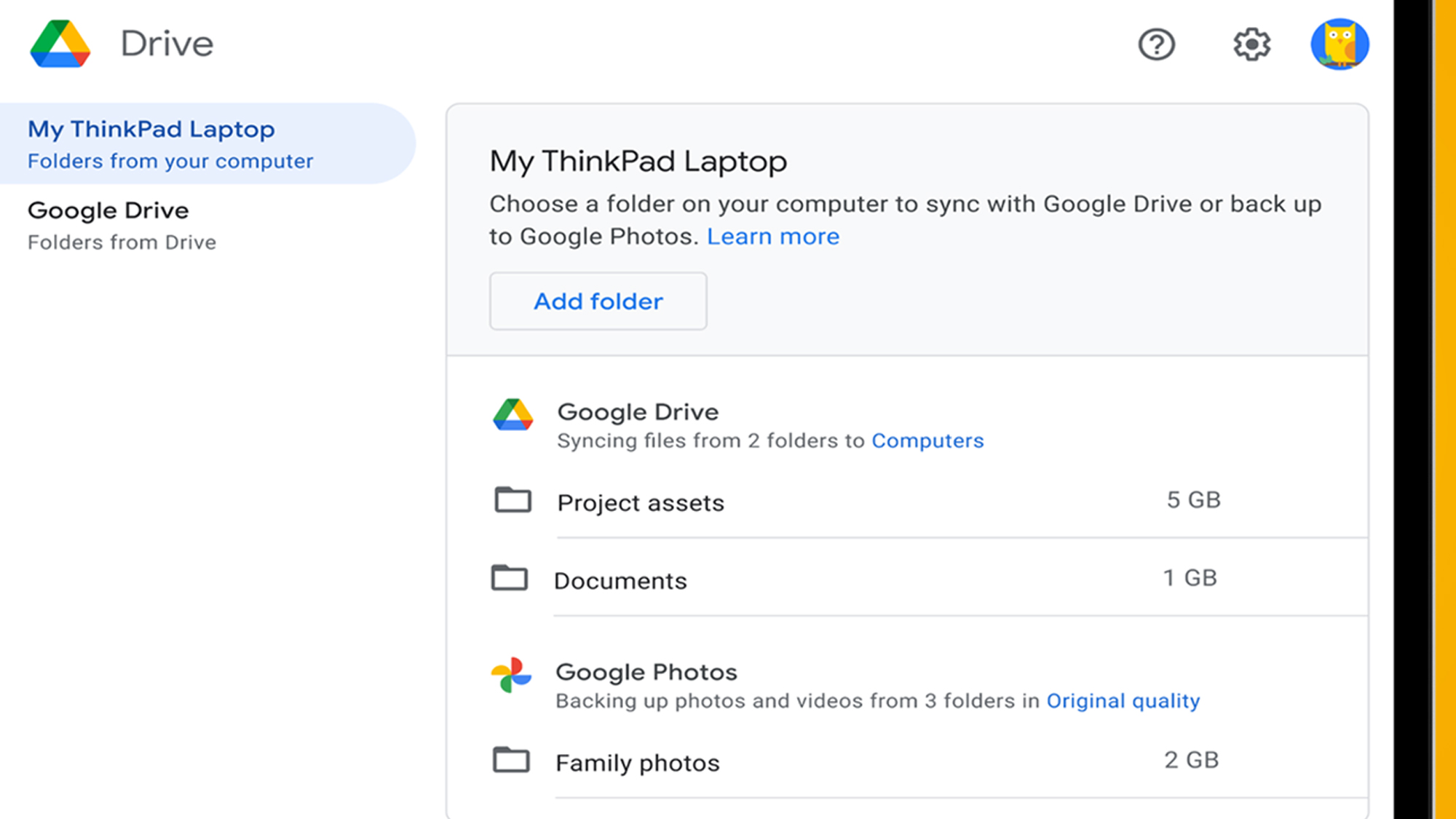This image depicts a screenshot of Google Drive's interface. In the upper left corner, the word "Drive" is prominently displayed next to the Google Drive logo, which is a triangle with green on the left, yellow on the right, and blue on the bottom. Below "Drive," there is a vertical menu listing several options. The first option is "My ThinkPad Laptop," followed by "Folders from your computer," which is highlighted in light blue, and "Google Drive," showing the associated folders.

On the right side of the window, the top section is labeled "My ThinkPad Laptop." Below this label, it prompts the user to choose a folder on their computer to sync with Google Drive or back up to Google Photos. An "Add Folder" button is present underneath this prompt. Further down, the section labeled "Google Drive" reveals storage usage: "Project assets" occupy 5 gigabytes, "Documents" use 1 gigabyte, and "Family photos" take up 2 gigabytes.